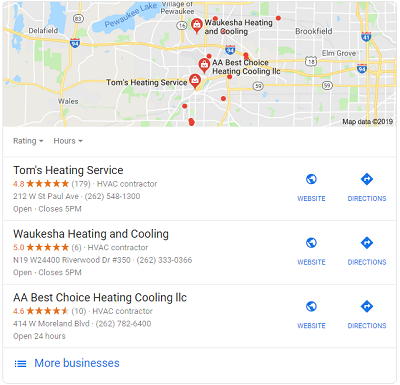This image is a screenshot of a Google search result page focused on HVAC contractors. The screenshot features a map at the top, pinpointing various service locations, though the specific city is not mentioned. However, the map includes an area labeled 'Brookfield.' Below the map, three highlighted search results are listed in detail:

1. **Tom's Heating Service**
   - **Rating:** 4.8 stars based on 179 reviews
   - **Type:** HVAC Contractor
   - **Address:** 212 West St. Paul Avenue
   - **Phone Number:** 262-548-1300
   - **Links:** Website and Directions
   
2. **Waukesha Heating and Cooling**
   - **Rating:** 5 stars based on 6 reviews
   - **Type:** HVAC Contractor
   - **Address:** N19-W24400 Riverwood Drive
   - **Phone Number:** 262-333-0366
   - **Links:** Website and Directions
   
3. **AA Best Choice Heating Cooling LLC**
   - **Rating:** 4.6 stars based on 10 reviews
   - **Type:** HVAC Contractor
   - **Address:** 414 W. Moreland Blvd
   - **Phone Number:** 262-782-6400
   - **Links:** Website and Directions

A thin gray line separates each business listing. Below these results, three horizontal blue lines and the phrase "more businesses" indicate additional options are available.